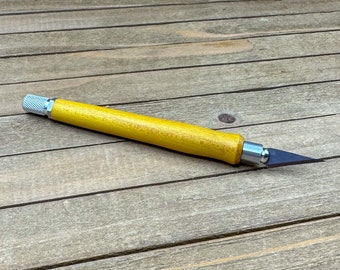The photograph showcases an X-Acto knife with a well-crafted, yellowish-tan, wooden handle that has been rounded for a comfortable grip. The handle is fitted with a textured, perforated metal cap, which features a twist mechanism allowing the user to tighten the inner sleeve that secures the blade. This sleeve is designed with a slot for the blade and is covered by an outer sleeve that, when twisted, causes the threaded rear handle to pull the tapered inner sleeve, effectively clamping the blade in place. The blade itself is long, sharp, and pointed. The knife is set on a background of unstained natural wood slats, adding a rustic touch to the scene with hues ranging from greyish to brownish shades. The entire knife appears to be a blend of stainless steel and wood with four primary colors visible: brown, grey, yellow, and black, with no text or markings except for a small dot on the handle.